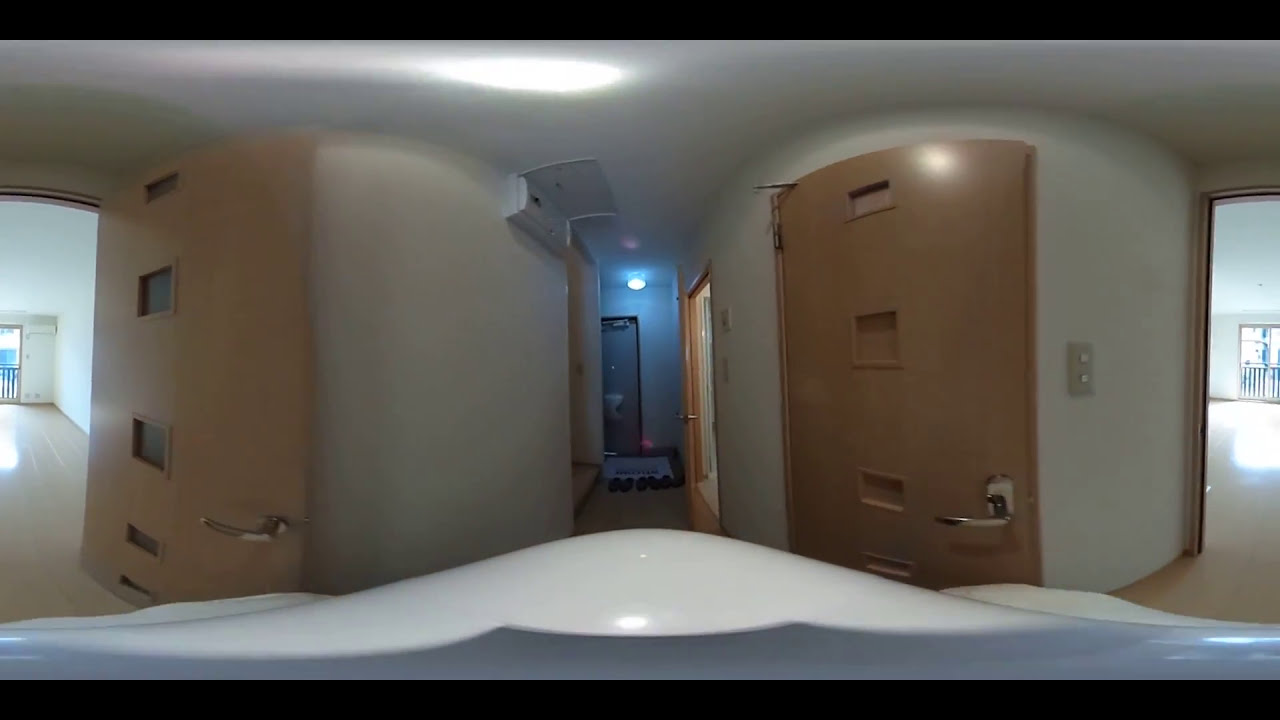The image depicts the interior of a possibly residential building, capturing a junction of several hallways. At the center is a small hallway, flanked by multiple doorways leading to different rooms. Directly ahead, there is another hallway extending toward us, ending in a door with an old piston stop at the top, suggesting it is a self-closing door. To the left, there is a wooden door that is open, revealing a short hallway with a window at the end, potentially looking out onto a deck with a railing. On the right side, another hallway is brightly lit with white light, also featuring a window and railing visible. The flooring appears to be hardwood, and the interior is lit naturally, indicating it might be daytime. The prominent colors in the image include black, white, gray, brown, light blue, dark gray, and a touch of red. The lack of any text and the detailed setting suggests the image was taken indoors, perhaps in someone's home, showcasing an area that includes light switches, air conditioning, and connected balconies.